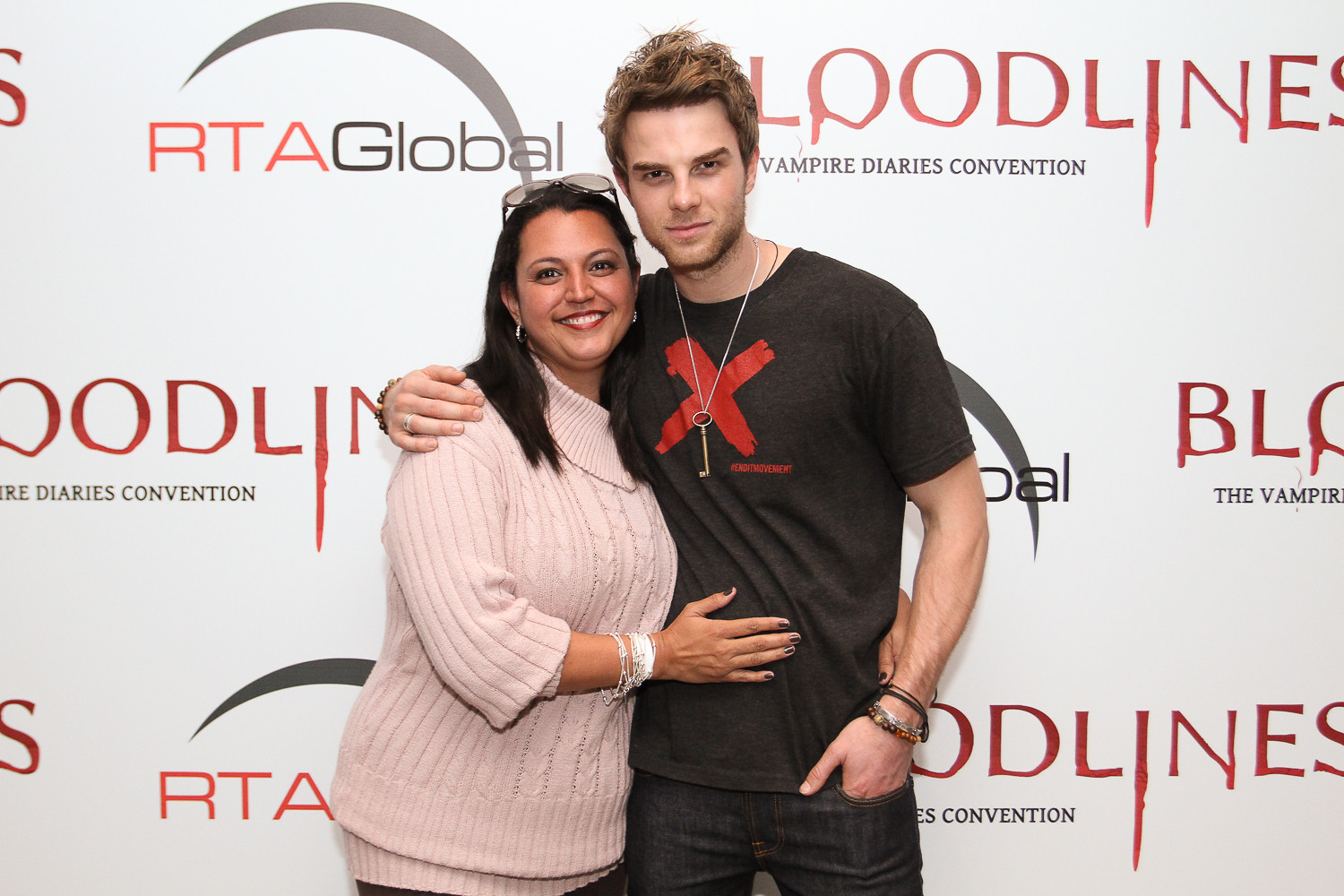In this detailed photograph, two people are posing in front of a backdrop typically seen at red carpet events, emblazoned with repeated logos that read "Bloodlines: The Vampire Diaries Convention" and "RTA Global." The word "Bloodlines" is strikingly written in dark red, with a font that appears to be dripping, evoking the image of blood.

On the left stands an Indian woman in her late 30s to 40s with shoulder-length, glossy black hair. She is dressed in an off-white or champagne-colored knit sweater and has a pair of glasses perched on top of her head. Her warm, engaging smile is directed at the camera as she leans slightly against the man beside her. Her hand gently rests on his stomach while her other arm is wrapped around his waist.

To her right is a younger white man, likely in his late 20s to early 30s. He is wearing a black t-shirt featuring a red X and has a key dangling from a necklace around his neck. The man has his arm around the woman, looking at the camera with a faint smirk, adding a hint of seriousness to his otherwise relaxed demeanor.